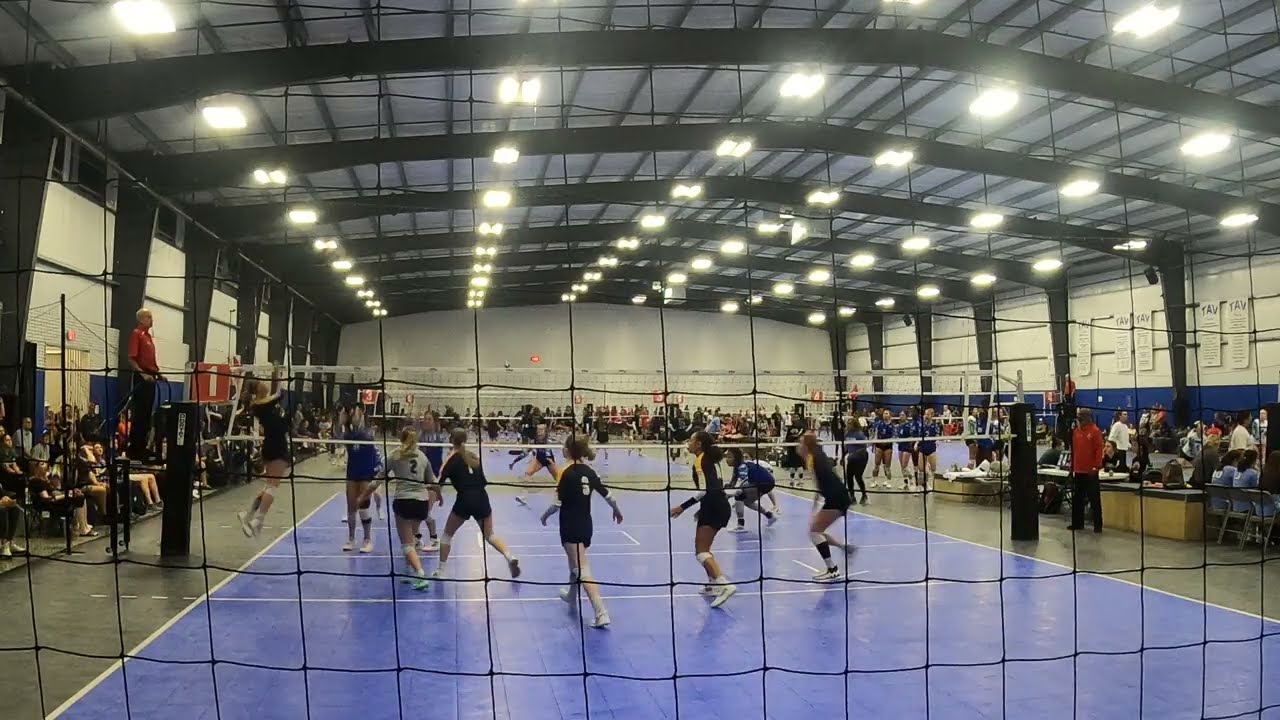The image depicts an indoor sports complex during a competitive girls' volleyball match. At the forefront, a player from one team, identifiable by their black jerseys, leaps into the air mid-spike, while a libero in a gray jersey can also be seen. The opposing team is wearing blue jerseys. The court features a gray and blue floor with distinct white boundary lines, and there is a volleyball net splitting the area. Positioned on either side of the court are referees in red shirts, overseeing the game. Spectators fill the stands on both the right and left sides, with the right side having bleachers likely occupied by parents or other supporters. Above them, the ceiling is dotted with numerous lights, dark-colored beams, and structural elements, and the white walls of the field house add a contrasting backdrop. In the distance, there are additional courts and ongoing games, indicating this might be a larger tournament setting. Notably, on the right side of the image, there are wood desks that could be for officials or judges critiquing the game. Overall, the scene captures the intense atmosphere of an indoor volleyball competition.